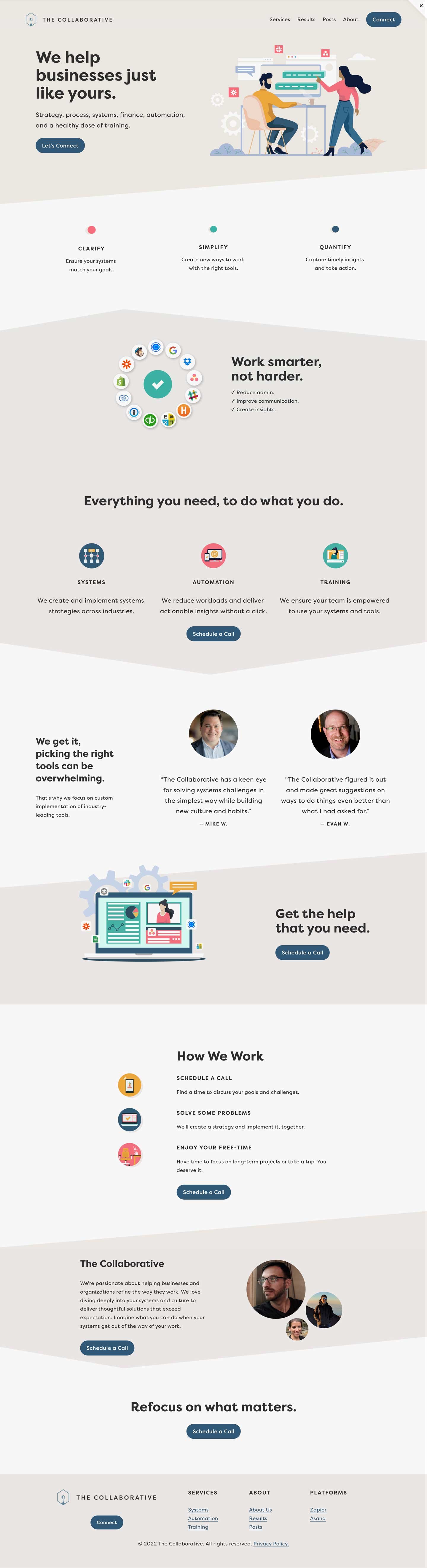A detailed caption for the described screenshot:

---

"This is a screenshot of an informational webpage from 'The Collaborative,' featuring a predominantly beige and gray background with alternating colored sections. At the top of the page, 'The Collaborative' is prominently displayed, followed by navigational sections labeled 'Services,' 'Results,' 'Posts,' 'About,' and 'Connect,' each highlighted with a blue pill-shaped icon. Below the header, a beige background bears the large text, 'We Help Businesses Just Like Yours,' followed by two lines of smaller, unreadable text. A button with the label 'Let's Connect,' also set on a dark blue pill-shaped icon, sits beneath this.

To the right, there's a clipart illustration of a man seated at a computer and a woman walking towards him, placing a teal line of text onto the screen. Below this, a gray section with an angular outline is divided into three parts: the left segment features a red dot followed by the word 'Clarify' and two lines of unreadable text; the center segment highlights a teal dot with the word 'Simplify' and two more unreadable lines; the right segment shows a teal or dark blue dot with the word 'Quantify' and two lines of text.

Beneath, a large beige area displays the phrase 'Work Smarter, Not Harder,' accompanied by three unreadable lines of text, each marked with a check. To the left, there is a teal circle icon with a white check mark, surrounded by various other icons arranged in a flower-like pattern. Below this, the statement 'Everything you need to do what you do' is visible. This structured, visually rhythmic design extends to the bottom of the extensive webpage."

---

This caption provides a comprehensive and detailed description, enhancing the user's understanding of the webpage's content and structure.